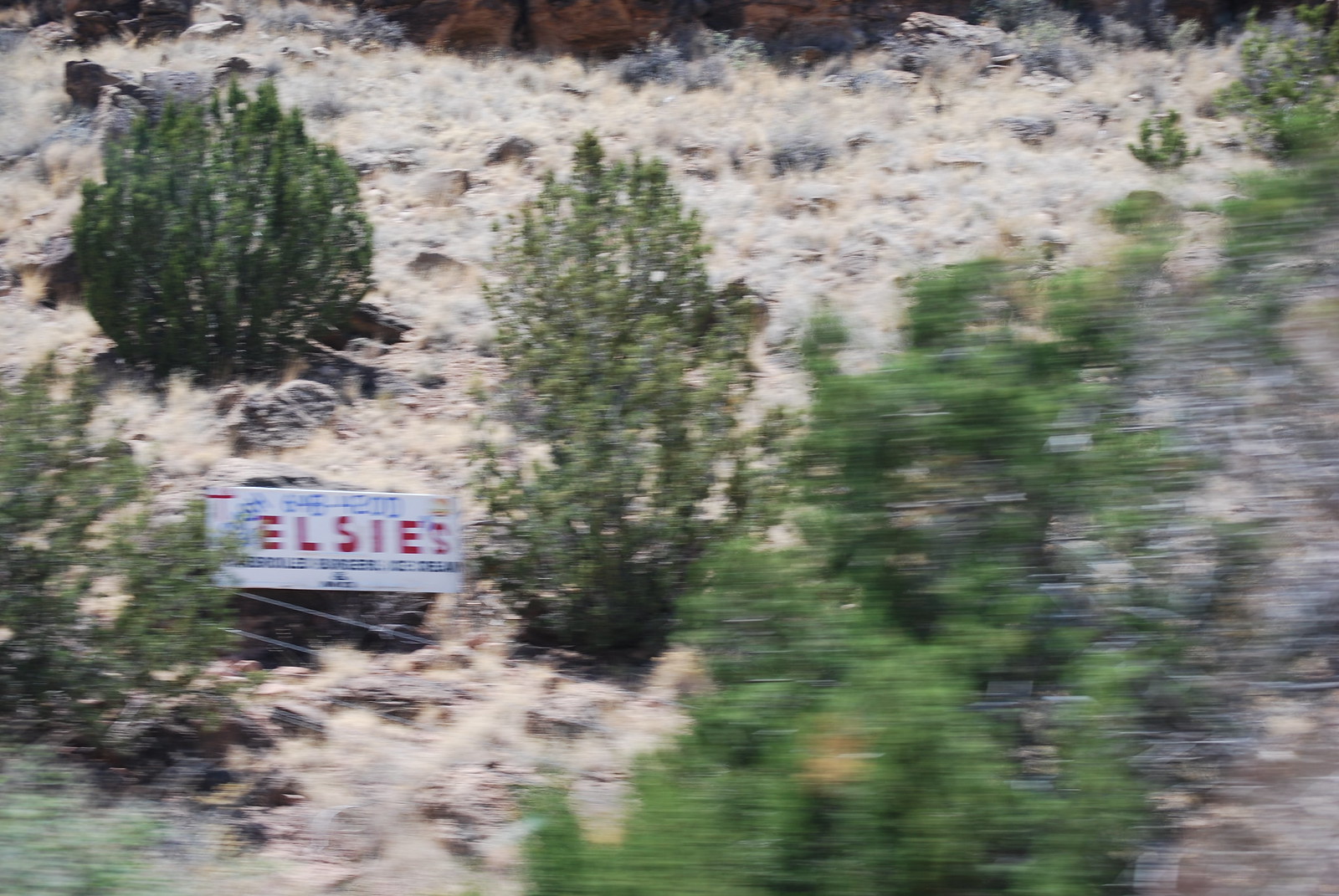The photograph captures a billboard situated on the side of a mountain, as seen from a moving vehicle. The image is slightly out-of-focus, adding a sense of motion and distance. Despite the apparent collapse of the metallic supports below, the billboard remains remarkably upright. The billboard's central text reads "Elsie's" in bold red letters, while additional, lighter blue text beneath is illegible due to the photograph's lack of clarity. Flanking the billboard are two trees, one on each side, providing a natural frame. The terrain at the mountain's top appears to be covered in either white foliage or possibly dead grass, suggesting a dry or wintry season. In contrast, the bottom left corner of the image showcases lush, green trees, adding a burst of color to the otherwise muted landscape.